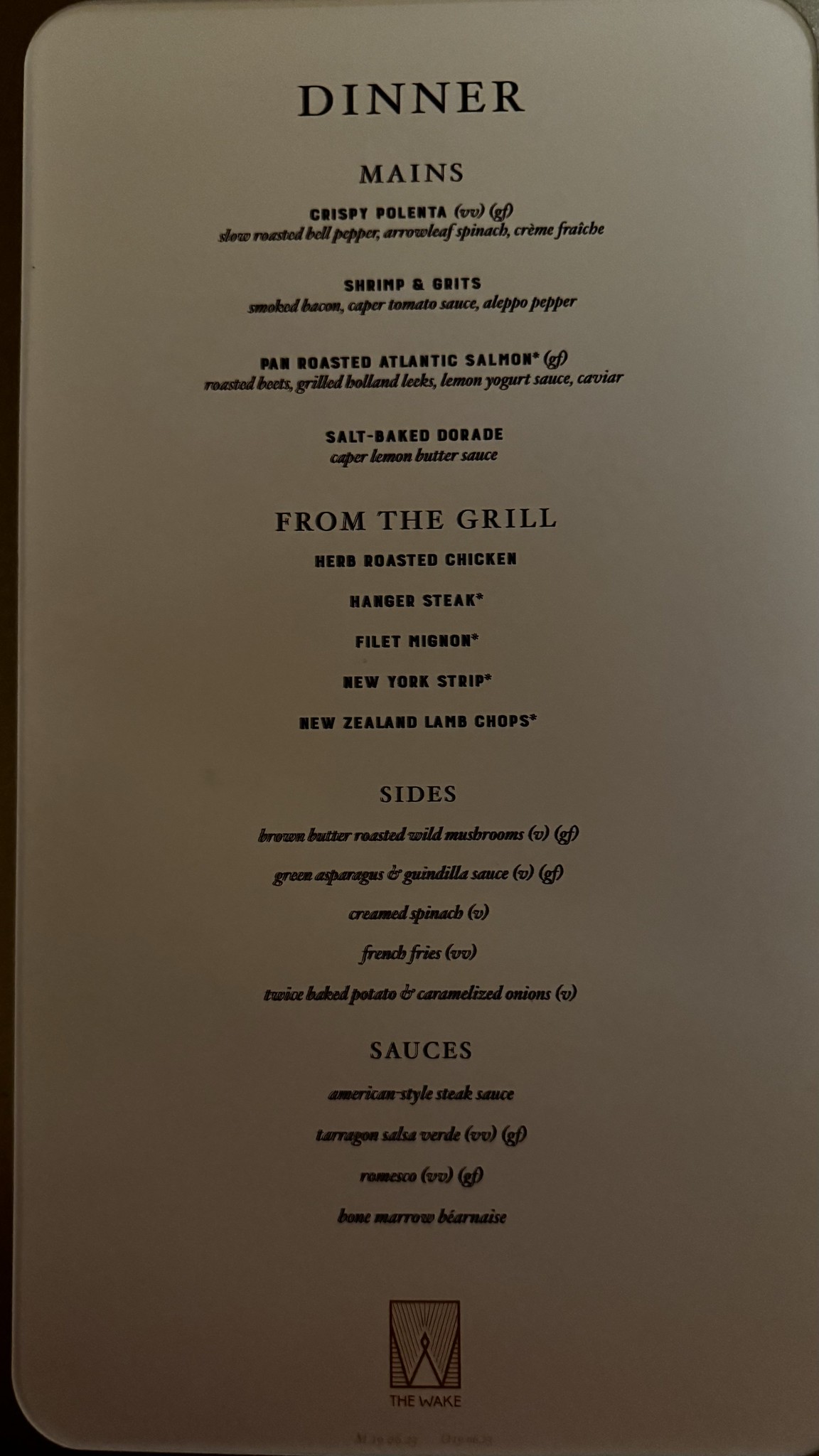This image features a detailed dinner menu with a clean, minimalist design. The menu itself is rectangular and has a white background with black text. At the top, it is prominently labeled "Dinner." 

Following that, the "Mains" section lists several enticing dishes:
- **Crispy Polenta** - accompanied by a description in elegant cursive writing.
- **Shrimp and Grits** - also detailed with a cursive description.
- **Pan-Roasted Atlantic Salmon** - described with cursive text.
- **Salt-Baked [Indistinct]** - partly obscured, but contains a cursive description.

Next is the "From the Grill" section, which features the following items without additional descriptions:
- Filet Mignon
- New York Strip
- Lamb Chops from New Zealand

The "Sides" section follows and includes:
- French Fries - with descriptions in cursive writing.
- Twice-Baked Potato with Onions - similarly detailed with cursive text.

The final section lists various "Sauces," though the descriptions here are harder to read due to the image's quality.

At the bottom of the menu, there is a logo that appears to be a square with brown writing, adding a touch of branding to the menu design.